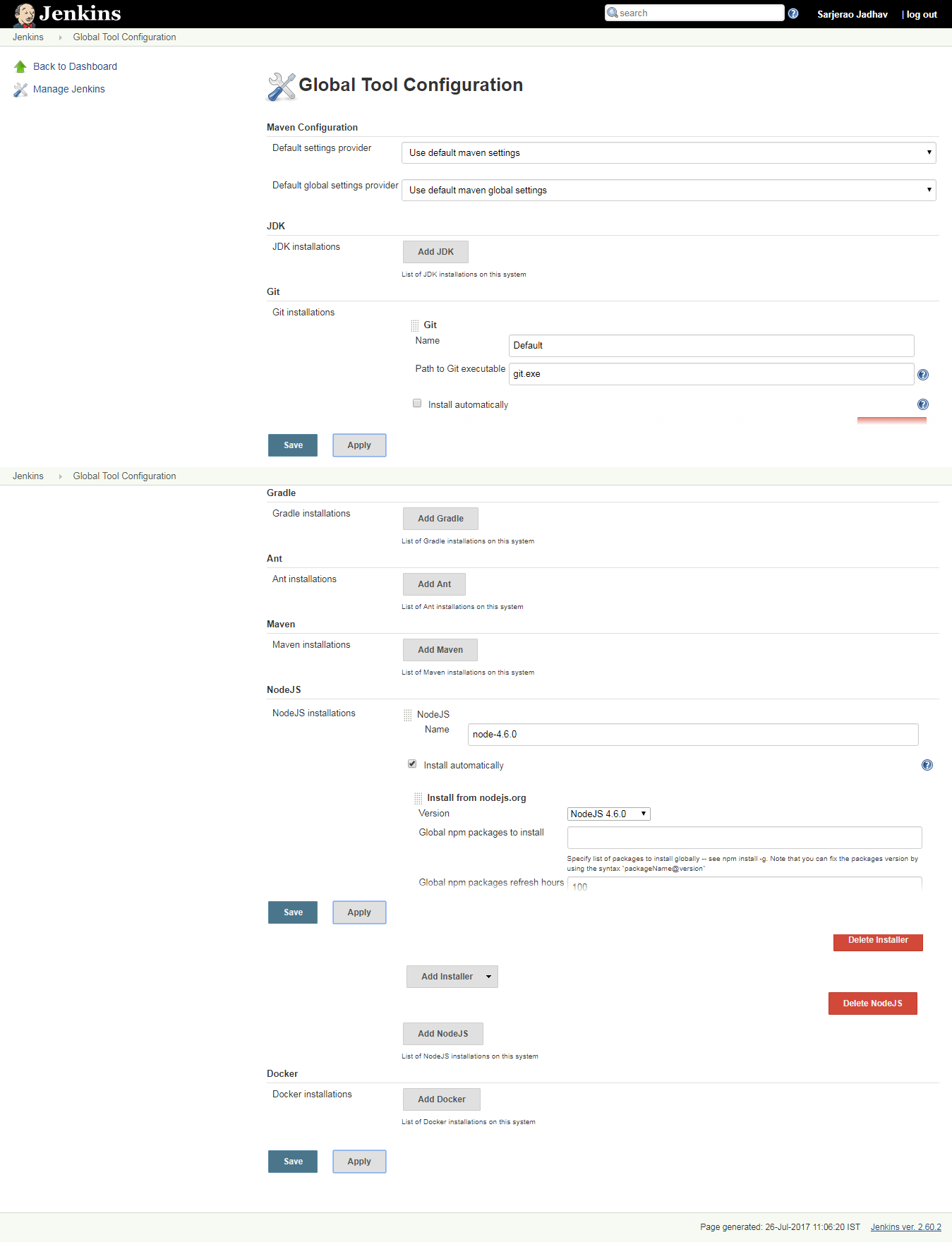This image depicts a zoomed-out view of a Jenkins web page with multiple options and sections. In the top-left corner, the word "Jenkins" is prominently displayed, and on the right-hand side of the header, there is a search bar accompanied by three small, barely readable white text elements. The main heading at the top of the page reads "Global Tool Configuration." The page is filled with text from top to bottom, which is too small to discern at this zoom level. 

In the top-left area, there are two menu options with drop-down arrows, as well as a gray rectangular button with another option, all requiring significant zoom to read clearly. Below these, there is a dark blue square containing an option, followed by a light gray square with another option. To the right, three more light gray squares each hold distinct options. Further down the page, there are two fields designated for information input. Additionally, the layout includes several more options within a couple of blue squares and five light gray rectangles. On the right-hand side of the page, two more rectangles with white text offer additional options. The entire page is set against a white background, providing a clean and organized, though currently unreadable, overview.